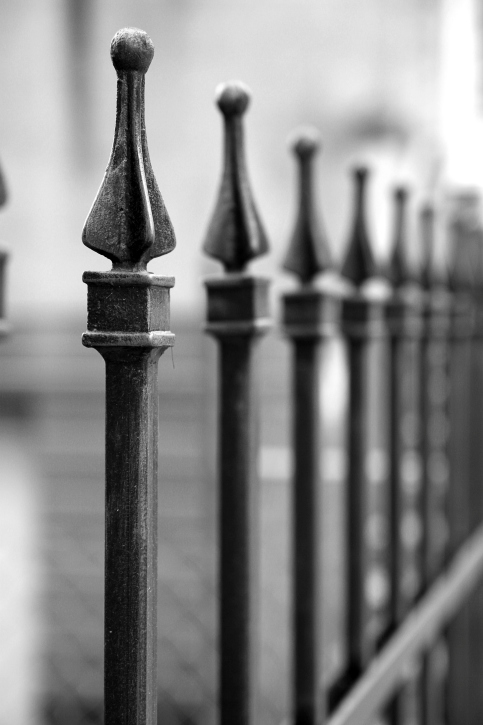This vertical black-and-white artistic photograph captures a focused, zoomed-in view of a large black wrought iron fence. The fence features long, vertical rods, each ending in a rounded, triangular shape or bulbous spike atop a square base. These rods are connected at various intervals by horizontal rods running from left to right. The sharp focus gradually softens, making the rods appear blurrier as they recede into the distance. In the background, an extremely blurry, indeterminate window or doorway provides a subtle hint of context without detracting from the primary subject. The stark contrasts created by the dark grays, blacks, and whites emphasize the intricate details and textures of the fencing.